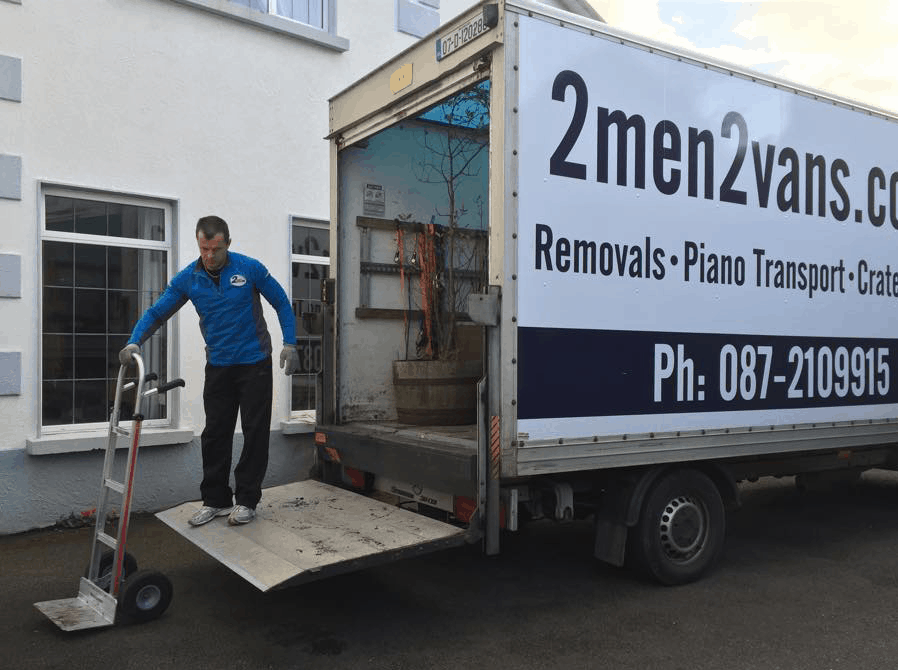The photograph, taken outside on a partly cloudy day, captures a dynamic scene under a vibrant blue sky with some clouds. Dominating the right side of the image is a large moving truck, its front part out of frame, with a white sign in black font that reads "2man2vans.com." Beneath that, the text advertises services like removals, piano transport, and crates, along with a phone number: 087-210-9915 in a black bar with white font. The truck is parked on asphalt in front of a building featuring large windows, hinting at a residential setting. A man wearing a blue shirt stands on the raised lift at the back of the truck, his hand resting on a hand cart. He appears to have just loaded a small tree in a pot into the truck. The moving truck's position on the right contrasts with the man and the hand cart on the bottom left, creating a balanced yet lively composition. The color palette includes blue, white, black, orange, red, and gray, adding to the image's vividness.